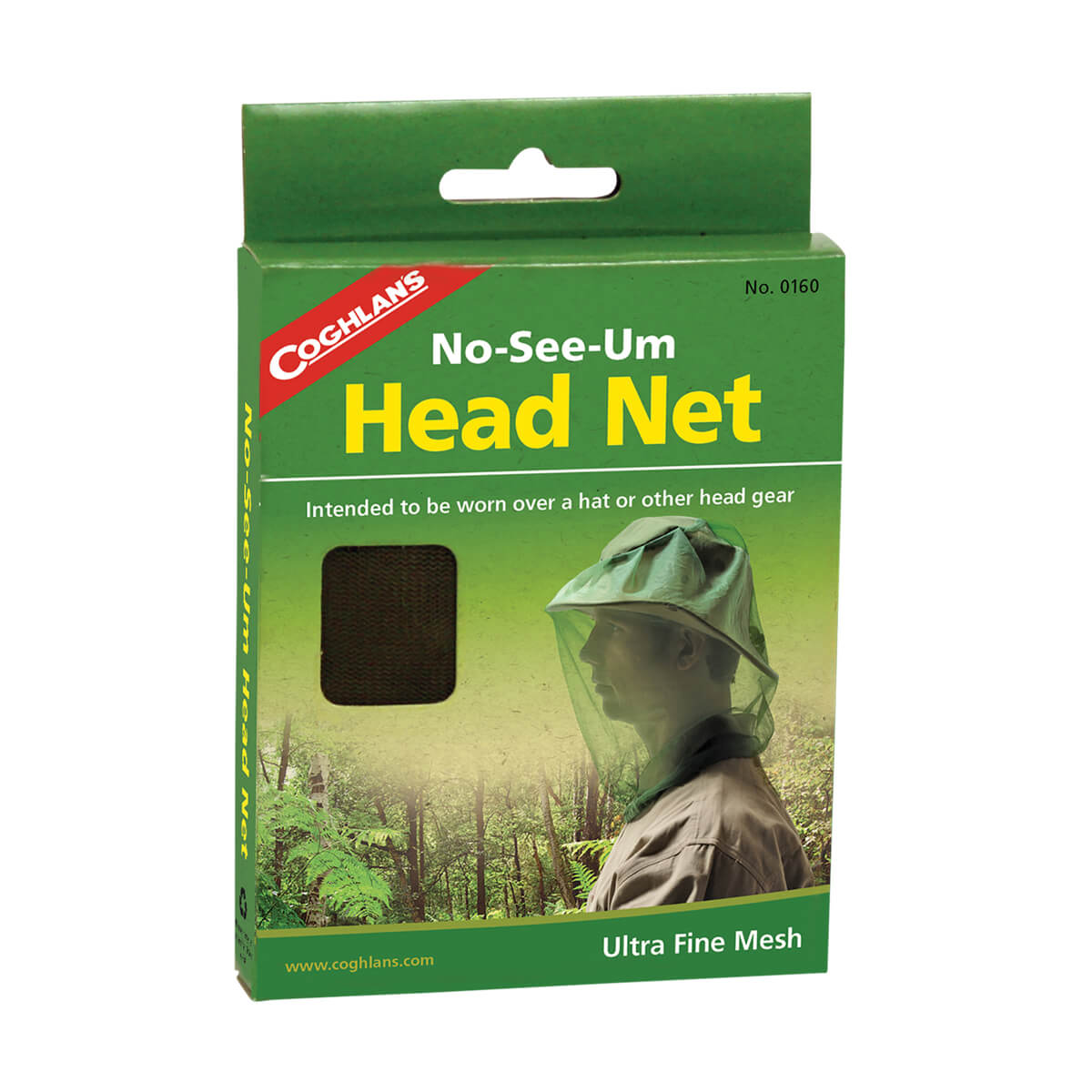The image depicts a rectangular green cardboard package for a product called the "Noceum Headnet" by the brand Coghlan's. The top part of the box features a handle with cut-out holes for hanging, and below the handle in the center, the words "Noceum Headnet" are prominently displayed with "Noceum" in white and "headnet" in large yellow letters. The product's number, "10160," is printed in small black text on the top right. A thin white line separates this information from an image of a man in a forest, wearing the headnet over a tan hat and green clothing. The headnet is designed to protect against tiny gnat-like insects known as "no-see-ums," and is made from ultra-fine mesh fabric, illustrated by a cutout showing the dark brown mesh material. The brand name "Coghlan's," spelled out in a white diagonal section at the top left, is accompanied by a red stripe. Additional text indicates that the headnet is intended to be worn over a hat or other headgear. The bottom of the package in a green stripe includes the website "www.coghlans.com" and the phrase "ultra-fine mesh" in white text. The left edge of the box repeats the product name and includes a recycling logo.